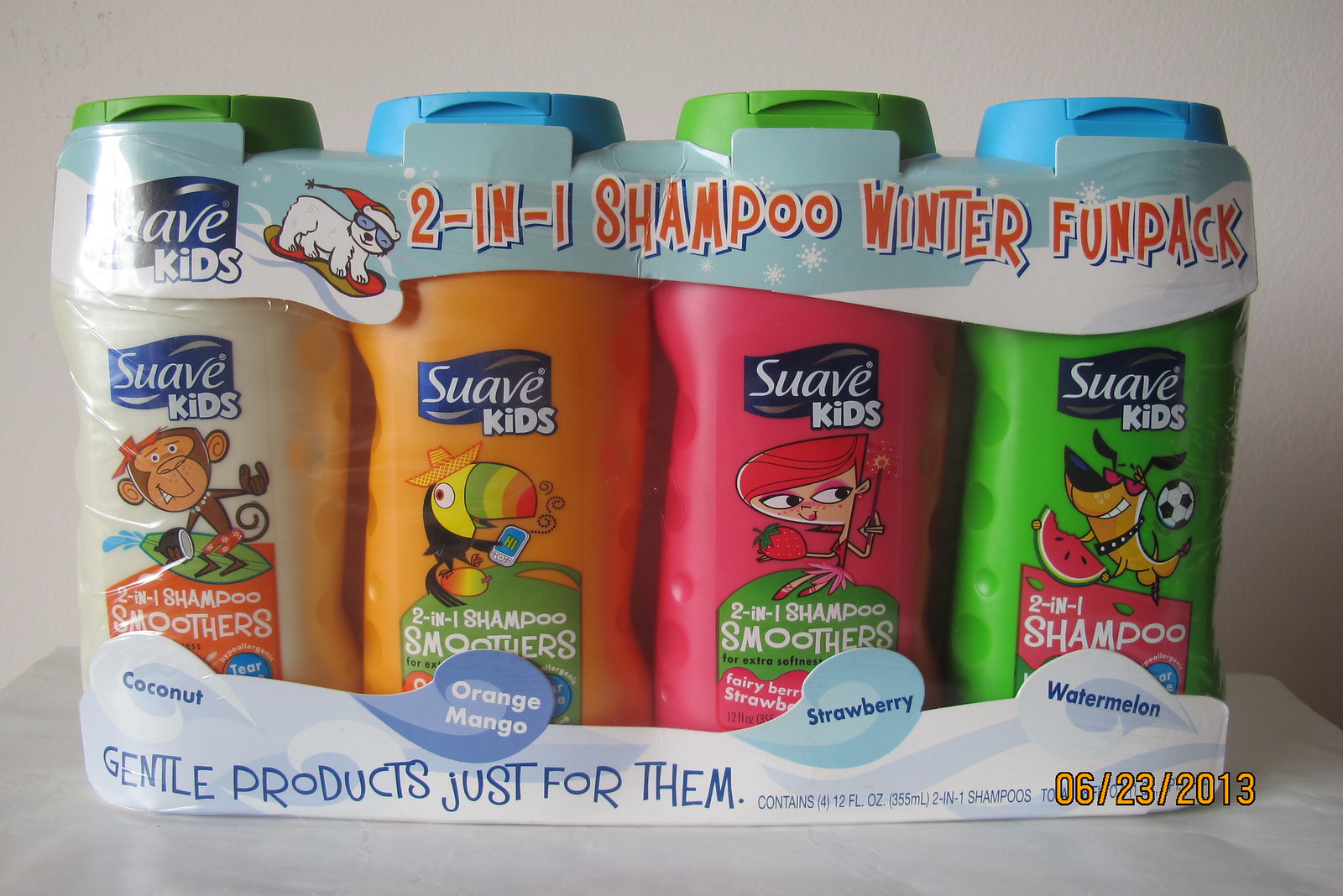This image is an advertisement for a Suave Kids Winter Fun Pack featuring four different Suave Kids two-in-one shampoo bottles, all wrapped together in clear plastic. At the top of the packaging, the Suave Kids logo is prominently displayed alongside an illustration of a bear snowboarding, wearing a red hat and sunglasses. The packaging also features the text "Two-in-One Shampoo, Winter Fun Pack."

Each bottle has a distinct design and flavor. The first bottle, with a green top and cream-colored body, features a monkey surfing with a coconut, labeled "Coconut." The second bottle, orange with a sky blue top, shows a colorful parrot in a sombrero and is labeled "Orange Mango." The third bottle, reddish-pink with a green top, has a fairy-like girl with pink hair holding a strawberry, labeled "Strawberry." The fourth bottle, green with a blue top, depicts a dog playing soccer and holding a watermelon, labeled "Watermelon."

The bottom of the packaging includes text that reads "Gentle products just for them," indicating the kid-friendly nature of the product. The scent labels at the bottom of the packaging reiterate the flavors: coconut, orange mango, strawberry, and watermelon. The image also includes a yellowish-orange digital timestamp reading "06/23/2013," suggesting the date the photo was taken. The background appears to be a beige bathroom wall, with a marble countertop beneath the package.